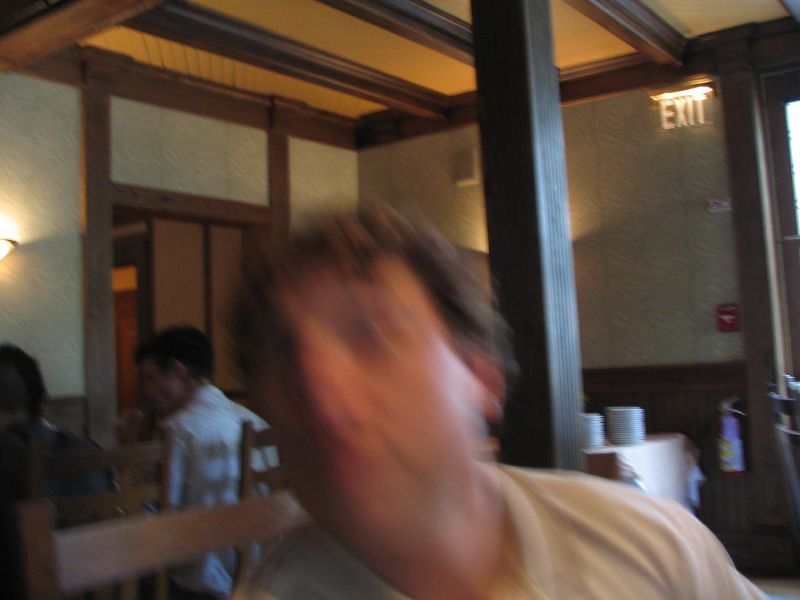In this photograph taken inside a restaurant, the primary subject in the foreground has a blurred facial effect, making it difficult to discern their features. The person’s light skin tone and short brown hair are faintly visible, and they are dressed in a tan-colored shirt. Sitting in a brown chair, this individual is placed prominently in front of a dark wooden post that extends up to the yellow ceiling, which is accented by dark wood rafter banisters. The restaurant's walls are adorned with gray, patterned wallpaper. Visible in the background, above a table with stacks of plates, are a fire alarm, a fire extinguisher, emergency lights, and a lit fire exit sign. To the left, a group of people sits, among them a noticeable person in a white shirt with short black hair. Additional people in both white and dark shirts are seated in brown chairs around the restaurant.